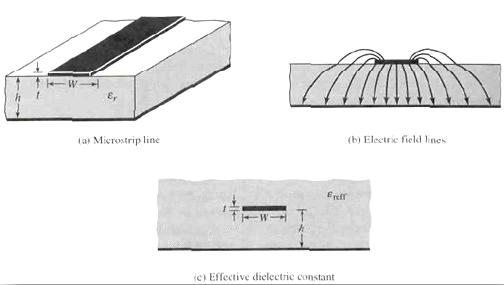The image is a black and white informational graphic presented in a landscape orientation with three distinct diagrams, two at the top and one below them. The top left diagram, labeled with the caption "Microstrip Line," features a white rectangular slab with a black stripe down the center. Dimensional notations such as H, T, W, and E subscript 'r' are indicated. To the right, a diagram labeled "Electric Field Lines" displays arrows curving from the edges of a smaller black rectangle towards a larger gray rectangle, forming a shape reminiscent of an upside-down bowl. The bottom middle diagram, captioned "Effective Dielectric Constant," shows a large gray rectangle again with dimensional notations H, T, W, and E subscript 'r', illustrating measurement attributes. Each diagram includes detailed annotations, emphasizing their educational and illustrative purpose related to electrical concepts.